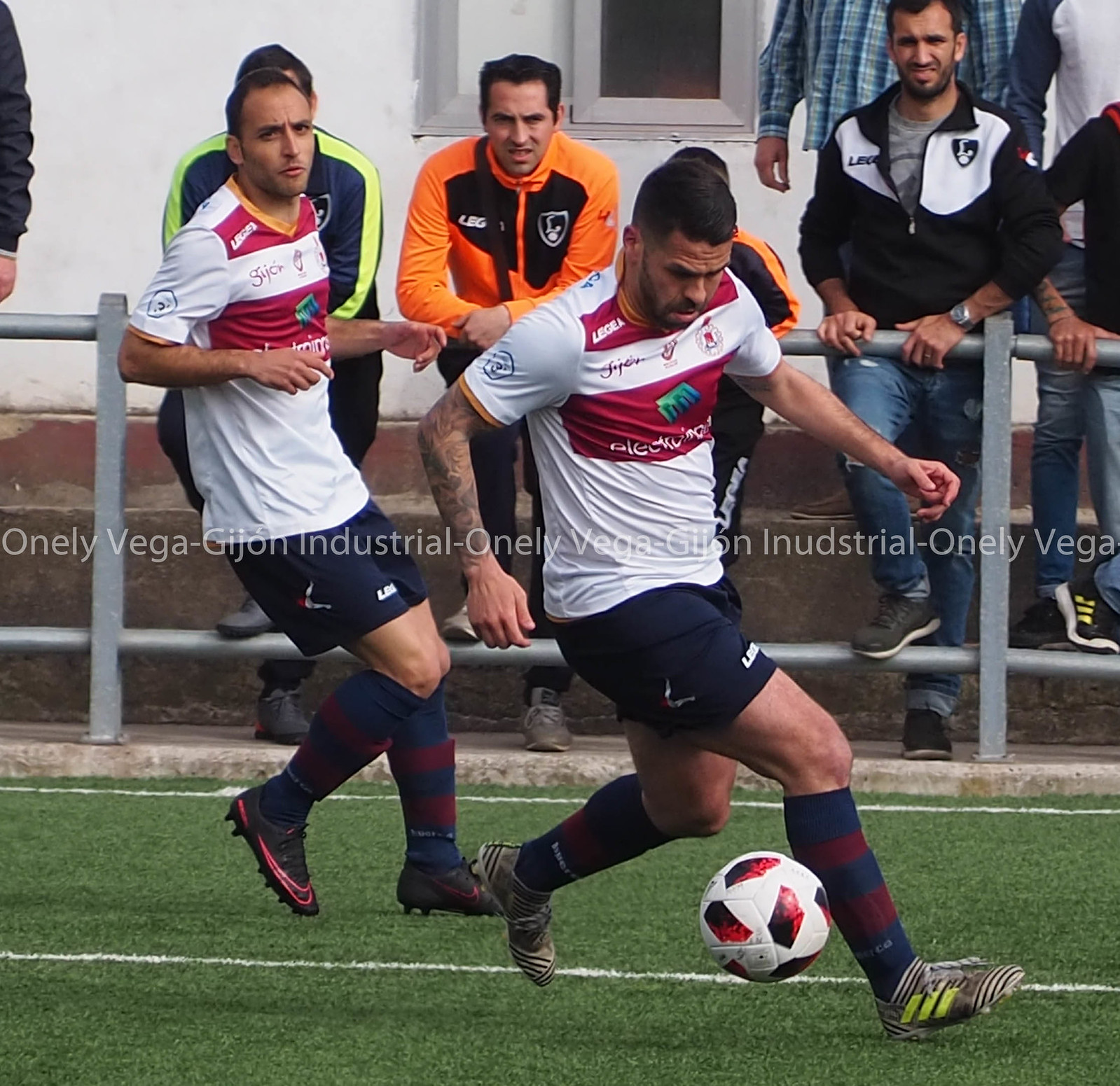In the image, a group of men are engaged in a lively soccer match on a lush green field. At the forefront, a white soccer ball poised for action catches your eye, with a man in a white jersey about to kick it. This player, dressed in dark shorts, blue and red striped socks, and tennis shoes, is slightly leaning forward, focused on the ball. A few steps behind him, another player in a similar white jersey with a red banner, dark shorts, and striped socks looks up, appearing to watch the ball closely.

Both players wear jerseys featuring small, unreadable logos and advertisements; one begins with an 'S,' and the red bar in the center of the jerseys bears more text that's difficult to decipher. The player further back appears to have dark hair and eyebrows, and like the man in the foreground, he is Caucasian with dark skin. 

In the background, separated from the field by a sturdy steel fence anchored by concrete pillars, several men observe the game intently. The spectators include a variety of individuals: one man in an orange outfit stands out in the center, flanked by a person in lime green and black on the left and another in a black and white jacket to the right. Additional onlookers include a man dressed in all black, one in a blue striped shirt, and another in a white jacket with dark blue sleeves, all wearing blue jeans.

Behind the spectators, a white wall with a brick bottom completes the scene. The atmosphere is framed by a white text overlay across the image that reads "one l y," followed by "vegas-gion" and "industrial," adding a somewhat surreal element to this dynamic sporting moment.